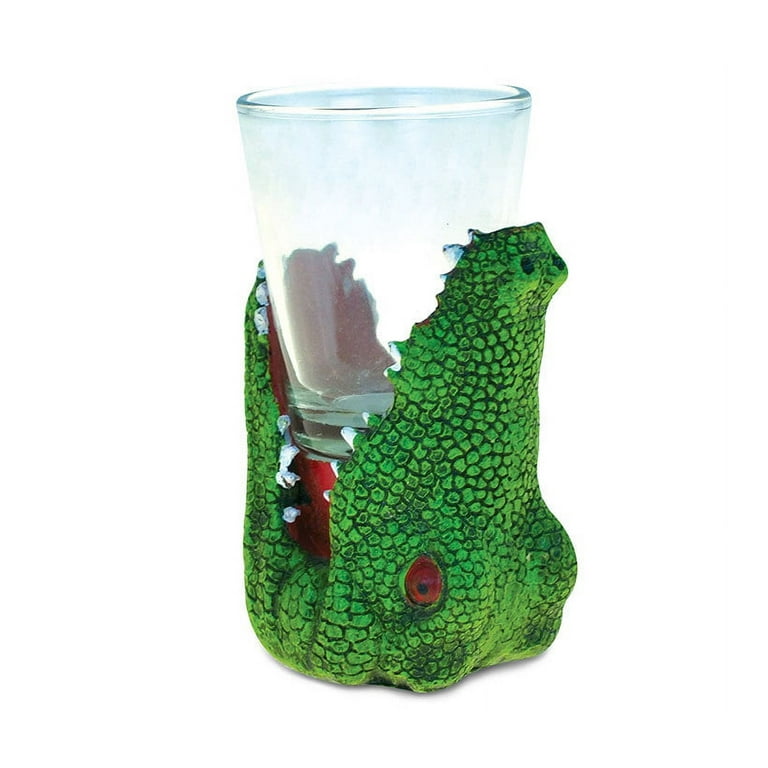The image depicts a unique and whimsical glass holder designed to look like the head of a crocodile. The crocodile is green with a distinct red eye and protruding white teeth. Its mouth is wide open, perfectly sized to grip and hold a clear, empty drinking glass within its jaws. The craftsmanship appears textured and detailed, pointing to a possible love for reptilian themes by its designer. The crocodile's head, positioned upside down, seemingly supports the glass against a white background, giving the impression it might be sitting on a table. This playful, eye-catching holder combines functionality with a fun and creative design, making it a standout piece.